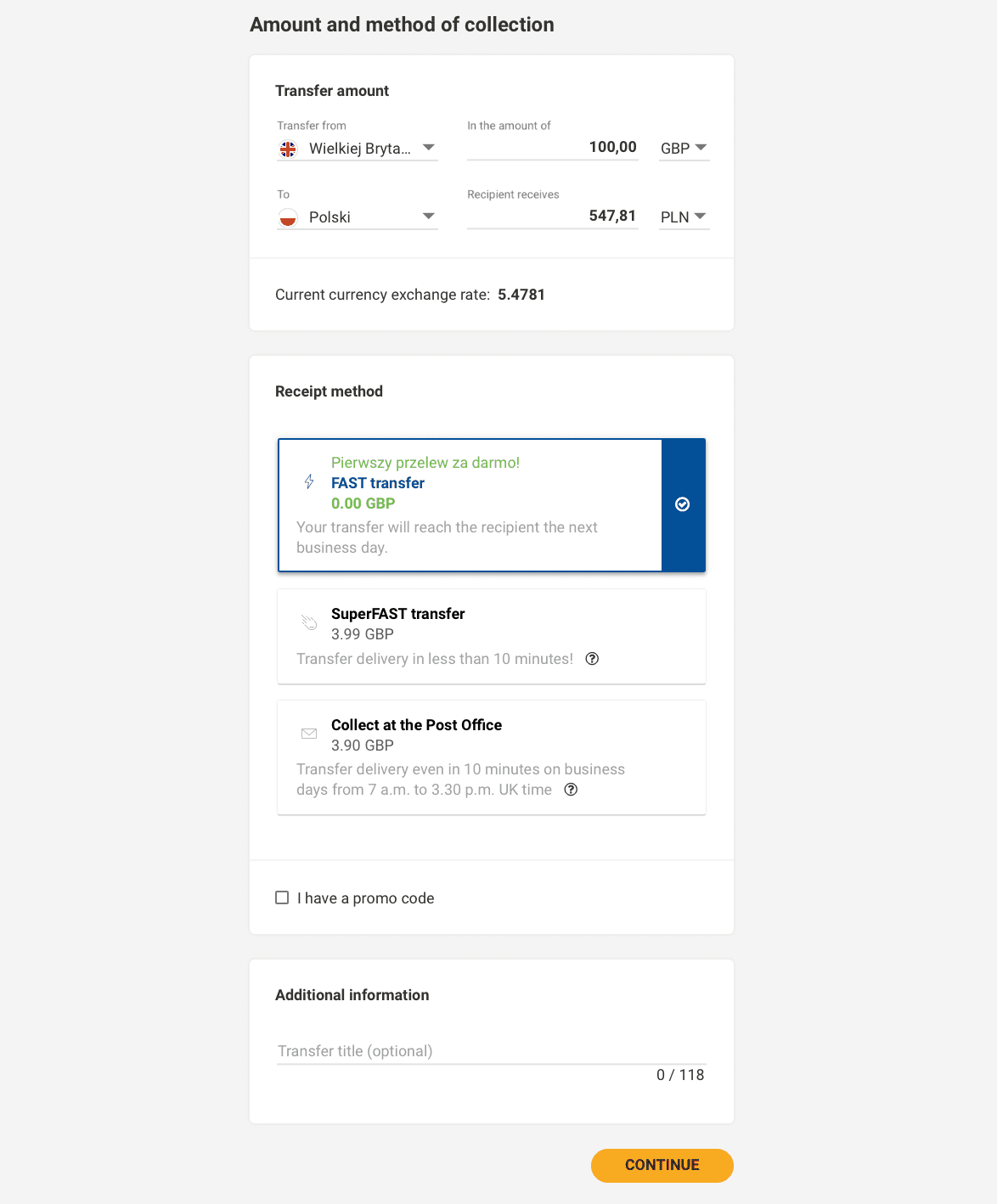This vertically oriented image appears to be a screenshot from a financial application on a smart device. The background is a flat, gray, one-dimensional design, free of any texture. At the top, the title "Amount and Method of Collection" is displayed in bold black text. Below this, there is a white text box.

Underneath the text box, additional black text reads "Transfer Amount Transfers From," followed by information translated from a different language. This information details a transaction involving a transfer of £100,000 GBP to "Poisky," and states that the recipient will receive 547,081 PLN (Polish Zloty). The current currency exchange rate is also provided, specified as 5.4781.

Further down, there is another white box labeled "Receipt Method." The content under this section indicates that the selected transfer method is "Per Whiskey Per Laws - Armom Fast Transfer" with no fee (0.0 GBP). It mentions that the transfers will reach the recipient the next business day. There are also two other unselected transfer options, and an option to click if you have a promo code. At the bottom of the screen, there is a section for additional information and a prominent orange "Continue" button.